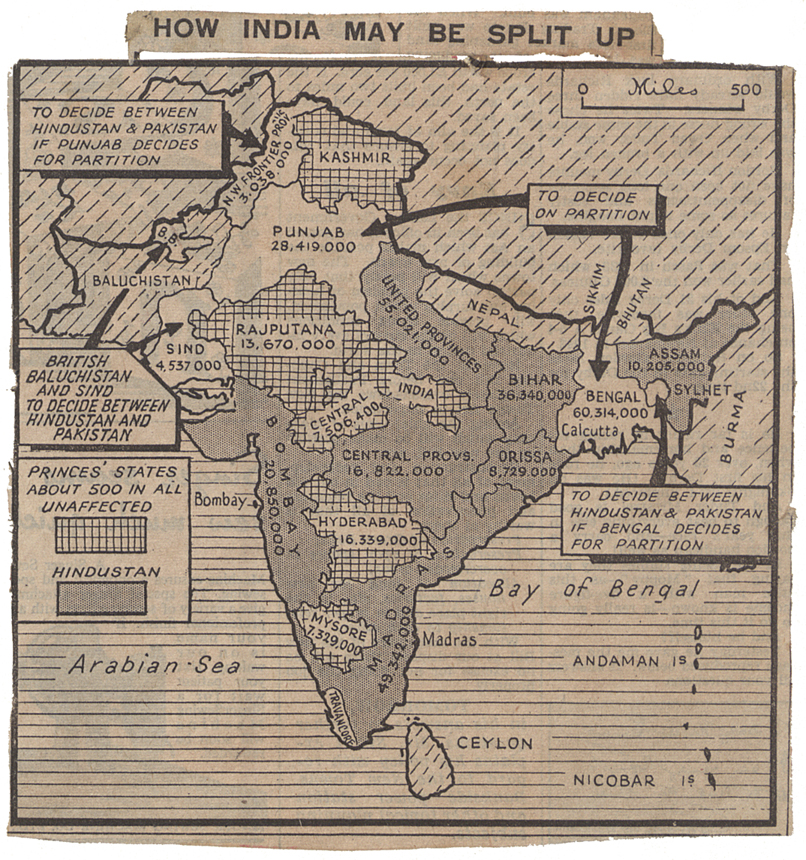This detailed, black-and-white map, possibly cut from an old newspaper, showcases a worn and frayed surface on tan paper with a distinct black border. The map captures a historical perspective on the potential partition of India, as indicated by the title at the top, which reads "How India May Be Split Up." Various regions and territories are labeled within the map, including Punjab, Kashmir, Bengal, Bombay, and others. Specific text boxes with arrows provide crucial detail, such as "to decide between Hindustan and Pakistan if Punjab decides for partition" and similar notes for Bengal, displaying the complex decisions involved in the partition. The top right corner features a scale running from 0 to 500 miles. The regions are color-coded, with Bengal and Punjab highlighted in white, while others are darker. Additionally, a legend in the bottom left corner explains cross-hatched areas as prince's states, which number around 500 and are unaffected by the partition. The Arabian Sea and the Bay of Bengal are marked, along with surrounding countries, including Burma and Bhutan, and islands like Ceylon, Andaman, and Nicobar.